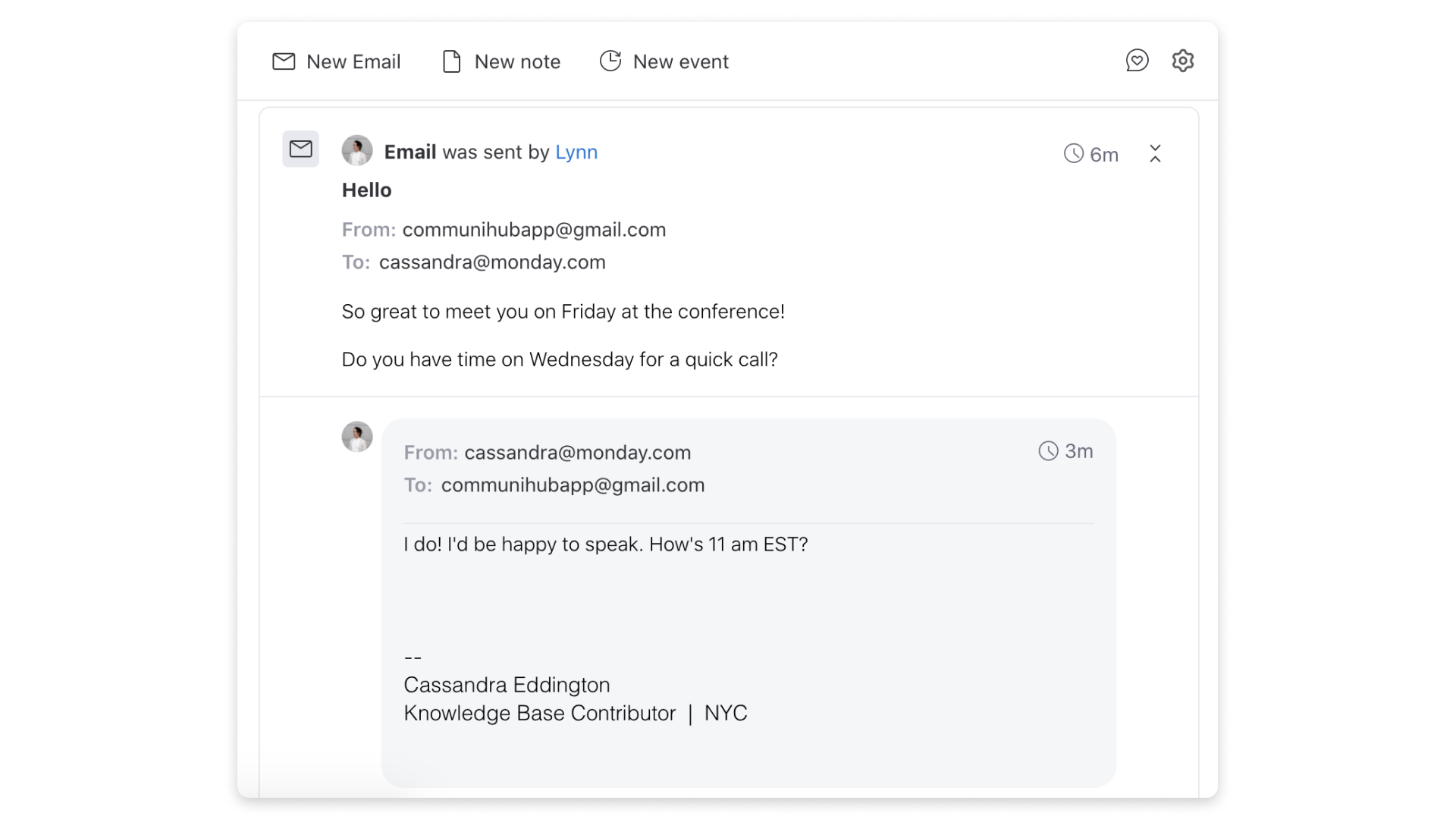The main section of the page features a white background. In the top left corner, there's a black outlined envelope icon accompanied by the text "New Email" in black. To the right of it, there's the outline of a page with its upper right corner folded inward, labeled "New Note." Further right, a refresh icon with a clock in the middle is paired with the text "New Event." 

On the far right corner, there's a chat bubble icon containing a heart outline in the center. Adjacent to this, a gear icon indicates settings. Below this top section, the background changes to light gray, although the main body of the image retains a white background.

In the upper left area of this section, a small gray square with a black email icon at its center is visible. To its right, there's a user icon depicting a male silhouette against a gray background. Further right, in bold black lettering, the word "Email" appears, followed by the gray, non-bold text "was sent by." Next to this in blue font, the name "Lynn" suggests a clickable link. 

On the far right, a gray clock icon is presented, accompanied by darker gray text reading "6M," indicating the email was sent six minutes prior. To the right of this, upward and downward arrowheads are shown for navigation.

On the subsequent line, bold black text reads "Hello," followed by smaller bold gray text "From:" and the email address "communihubapp@gmail.com" in black.